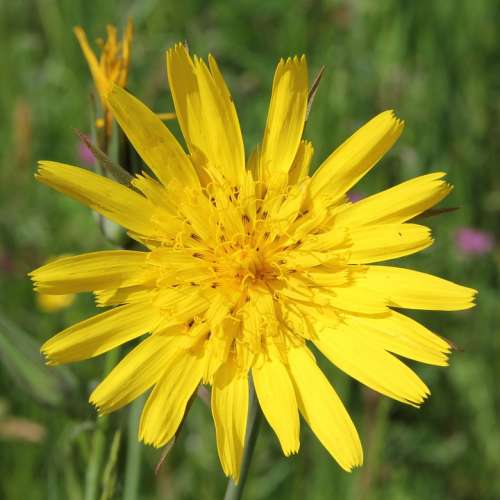In the image, a vibrant yellow flower is fully in bloom, showcasing its many elongated petals that taper into four to five distinct points, resembling a crown. The flower's center is a prominent circle with hints of orange, indicating where seeds will form. The thin, dark green stem supports the flower, while a similar, yet-to-bloom flower is visible in the background. The scene is set in a sunny field, with green vegetation and blurred purple and pink flowers adding a soft, colorful contrast. The overall background appears fuzzy, enhancing the focus on the yellow flower and giving a sense of a warm, sunlit day.